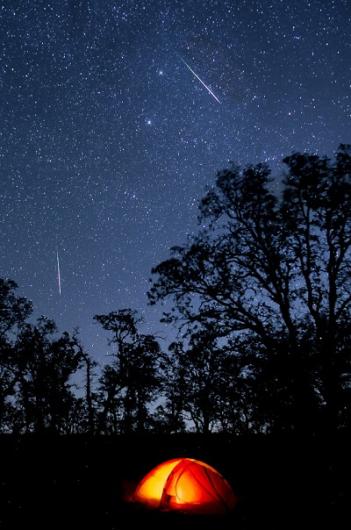The image captures a serene nighttime scene set in the woods. The dark blue sky, studded with countless stars, including several brighter ones and at least two visible shooting stars, serves as the stunning backdrop. Silhouettes of treetops, possibly oak trees, create a delicate outline against the starry expanse. The bottom of the image is shrouded in darkness, highlighting the glowing light from within a small, domed tent. This tent, with its inviting orange and yellow radiance, forms the focal point of the image, standing out vividly against the otherwise tranquil and dark surroundings.